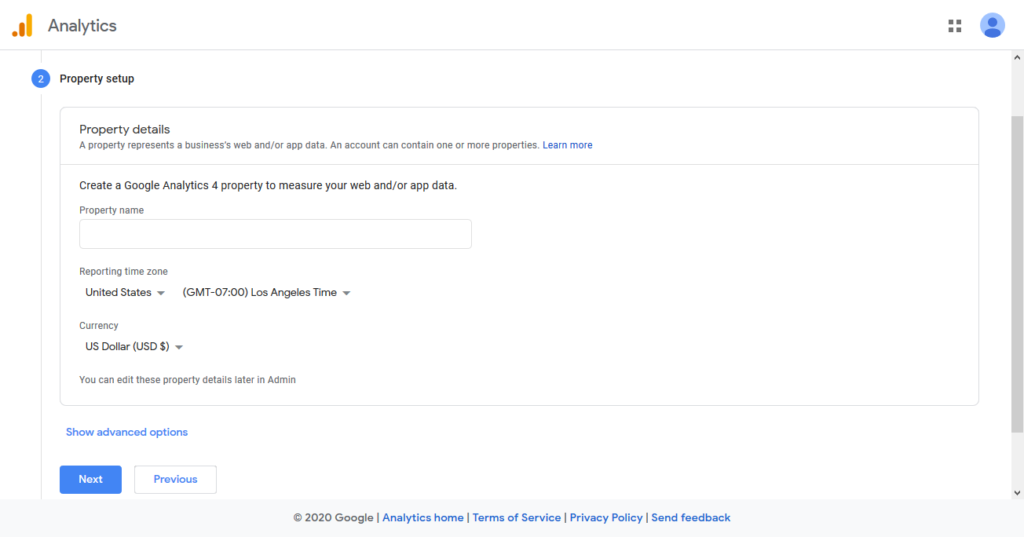Screen Capture of a Google Analytics Property Setup Page

This screen capture showcases a Google Analytics application interface centered on the setup of a new property. The interface invites the user to create a "Google Analytics 4 property" to gather and measure web and/or app data effectively. Essential configuration details are highlighted, including:

1. **Property Details**: 
   - **Property Setup Instructions**: A prompt guides users through the initial setup steps.

2. **Settings**:
   - **Location**: The default setting is configured for the United States.
   - **Time Zone**: The time zone is set to Los Angeles time.
   - **Currency**: The currency is indicated as US Dollar (USD).

3. **Navigation Options**:
   - A "Show advanced options" link is available for additional configuration choices.
   - Navigation buttons labeled "Next" and "Previous" help users move through the setup process.

4. **Footer Information**:
   - **Copyright Notice**: © 2020 Google
   - **Links**: Quick links to the Google Analytics home page, terms of service, privacy policy, and a feedback form are provided.

Overall, this screen capture captures the essential elements involved in setting up a new property within the Google Analytics application, facilitating users to efficiently measure and analyze their web or app data.